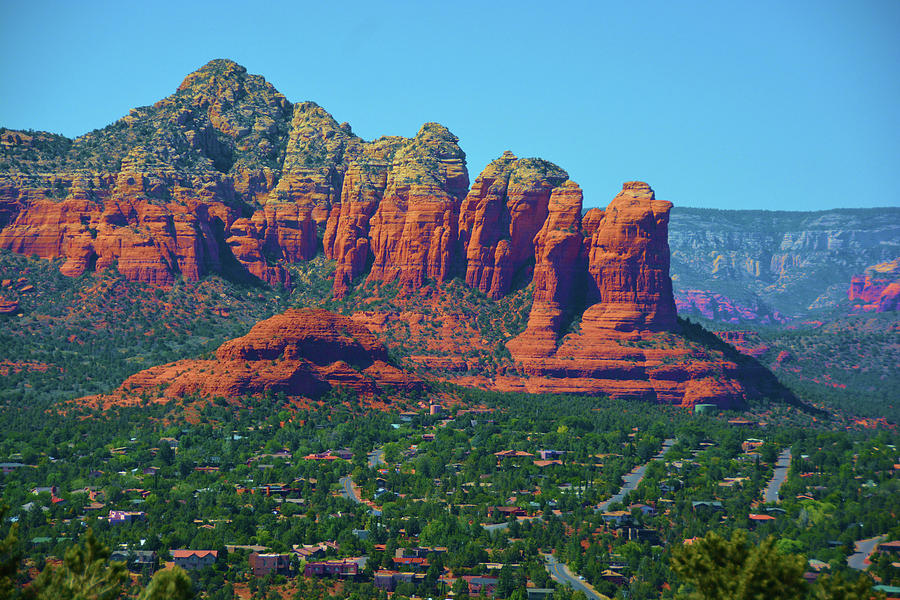This outdoor photograph captures a vibrant landscape that appears to be either the Badlands or some canyons. The foreground is dotted with numerous bright green trees, amidst which small houses are scattered, connected by pockets of dark gray roads. The middle section features grand, clay-colored rock structures, with some transitioning into a richer brown hue, and others displaying a darker green at their tops. As the eye moves further into the background, these rock formations shift to various shades of gray and red, particularly on the right-hand side. The entire scene is set against a brilliant, turquoise-blue sky, adding an energizing and somewhat surreal quality to the overall image.